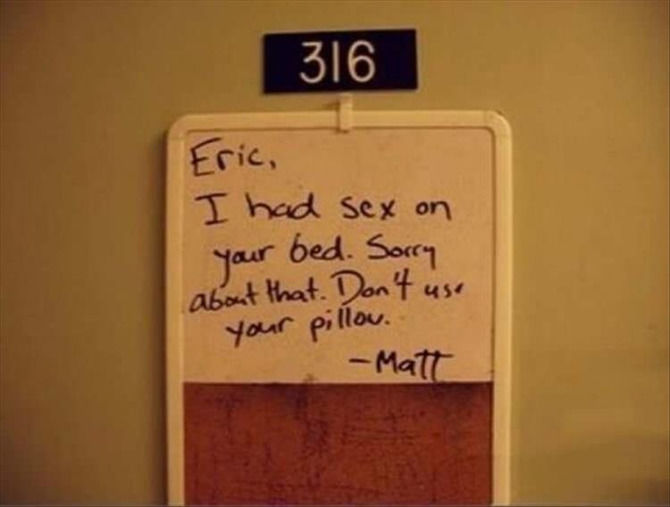The photograph depicts a close-up view of a yellowish-brown door, likely that of a dormitory room, with key identifiers situated centrally near the top. The main features include a small black placard with the room number '316' in white font. Directly beneath this is a rectangular message board, edged in white. The upper portion of this board is a dry erase surface featuring the handwritten message in dark blue or purplish ink: "Eric, I had sex on your bed. Sorry about that. Don't use your pillow. Matt." The bottom section of the board appears to be a cork material but remains unoccupied. All elements in the image are in an upright position, and no further text is present.